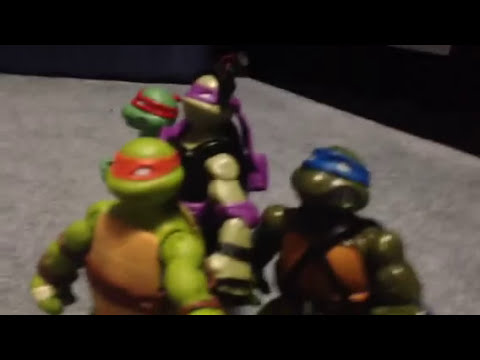The image depicts a blurry and poorly lit scene featuring figurines of the Teenage Mutant Ninja Turtles, likely positioned on a gray surface that resembles asphalt or a tabletop. The camera view is slightly rotated to the left and elevated about 6 inches above the heads of the characters, angled downward. There are four Ninja Turtles in the picture, facing slightly left and looking off into the distance. 

In the bottom left corner, there is a light green turtle with an orange bandana and light brown chest padding. To the right, another light green turtle stands in the center, wearing a purple mask and a black suit. To the left of this central turtle, a dark green character with a blue bandana and a hint of a black and brown suit is visible. Additionally, in the bottom right corner, another dark green turtle appears with a red bandana. In the background, they are placed against a gray surface with black walls and strips framing the top and bottom of the image. The poor image quality and lighting make it difficult to discern much more detail, but the general arrangement and uniforms of the characters are clear.